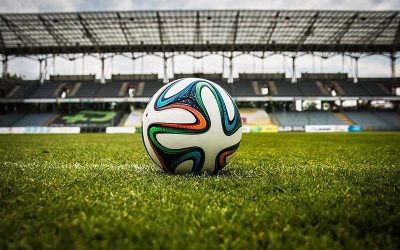This photograph features a close-up view of a distinctive soccer ball placed on a vibrant green turf field within an empty stadium. The soccer ball itself is predominantly white and adorned with intricate designs in blue, green, black, and orange, reminiscent of a Triskelion pattern, with the colors forming curved shapes around its surface. 

The grass underneath the ball is lush and bright, adding to the vividness of the image. In the blurry background, the stadium seats appear gray, with no spectators present, suggesting a calm and unoccupied setting. There is a partially covered structure overhead, with a cantilevered roof and white sky visible through the open back of the stadium, evoking a blue and slightly cloudy day. 

The overall composition highlights the soccer ball as the focal point, with an empty field and out-of-focus seating areas providing context to the sporting location. Minimal details such as some distant advertising and a black netting panel are also visible but do not detract from the central subject.